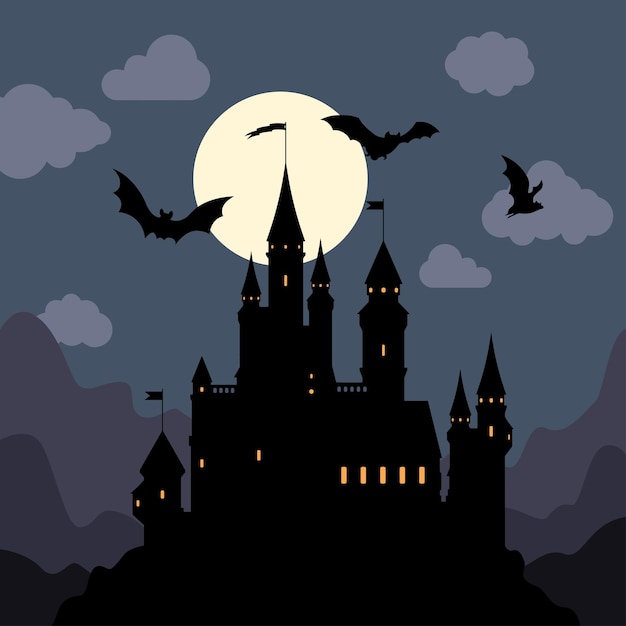The image depicts a hauntingly beautiful, night-time scene of a silhouetted, black castle perched atop a hill. The castle features eight towers of varying heights, three of which are adorned with black flags: one on the highest tower, one on the lowest tower to the left, and another two towers to the right of the highest point. The numerous windows of the castle emit an eerie yellow glow, piercing through the dark façade. Surrounding the castle, three bats are silhouetted against the night sky, which is a deep blue. The sky is dotted with light blue-gray clouds. In the background, behind the castle, are mountains painted in shades of black and purple. A large, round, white moon looms directly behind the tallest tower, further accentuating the mysterious atmosphere of the scene.